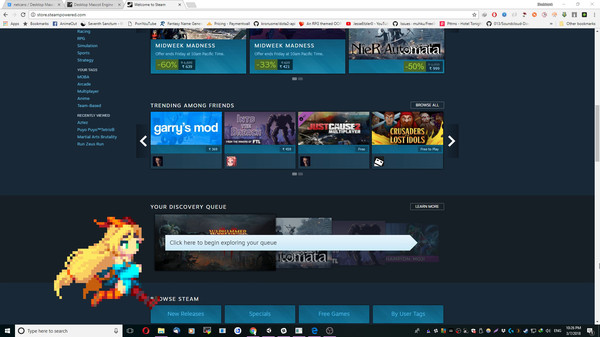Screenshot captured from a website's interface. At the top, three prominent rectangular banners are displayed, each containing specific information: the first two banners announce "Mid-Week Madness," while the third highlights "Naira Asatika." Below these, a row is labeled "Trending Among Friends," showcasing popular games such as "Gary's Mod," "Just Cause," and "Crusader's Lost Idols." At the bottom of the screenshot, there is an image of a young girl running towards the right, set against a vibrant background. Adjacent to the girl, an arrow points towards a button labeled "Click Here to Begin Exploring Your Queue," referring to the user's discovery queue. Additionally, a browse stream menu lists categories such as "New Releases," "Specials," "Free Games," and a section titled "By User Tags."